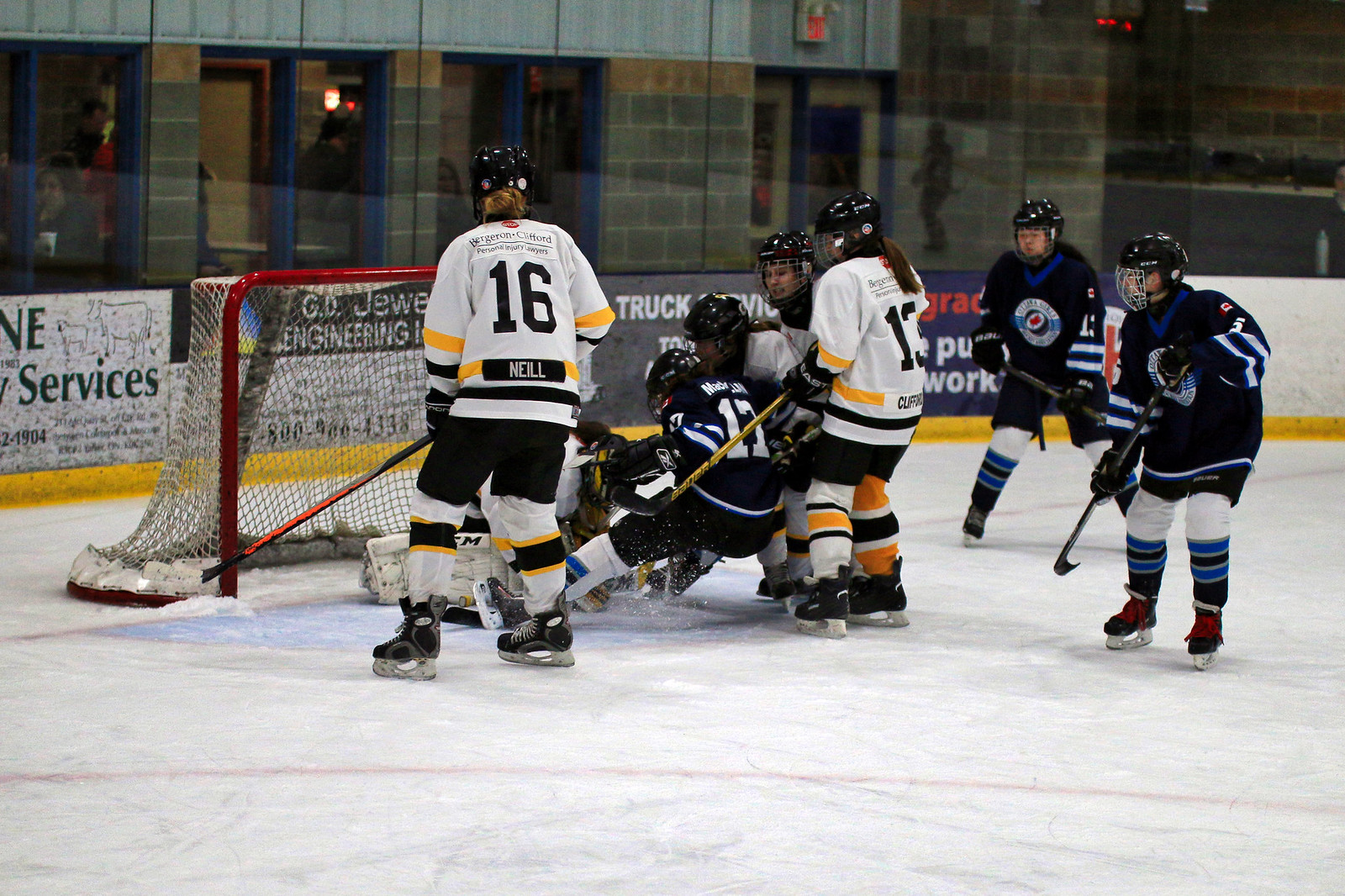This image vividly captures a dynamic moment in a women's ice hockey game taking place in a brightly lit arena. The two teams are distinguished by their uniforms—one team is clad in white jerseys with black and gold trim and dark pants, while the opposing team wears black jerseys with white and blue stripes. The action is centered in front of the goal, where players from both teams are fiercely battling for control of the puck. Notably, a player on the black team, wearing the number 17 jersey, is being pulled down amidst the chaos. The tension of the game is palpable as others cluster tightly around, leaving little open ice in front of the net. Surrounding the rink, the boards are adorned with various advertisements, though the space behind them appears empty, lacking spectators. In the background, the natural light highlights some stone structures and an emergency exit, adding to the arena's atmosphere.